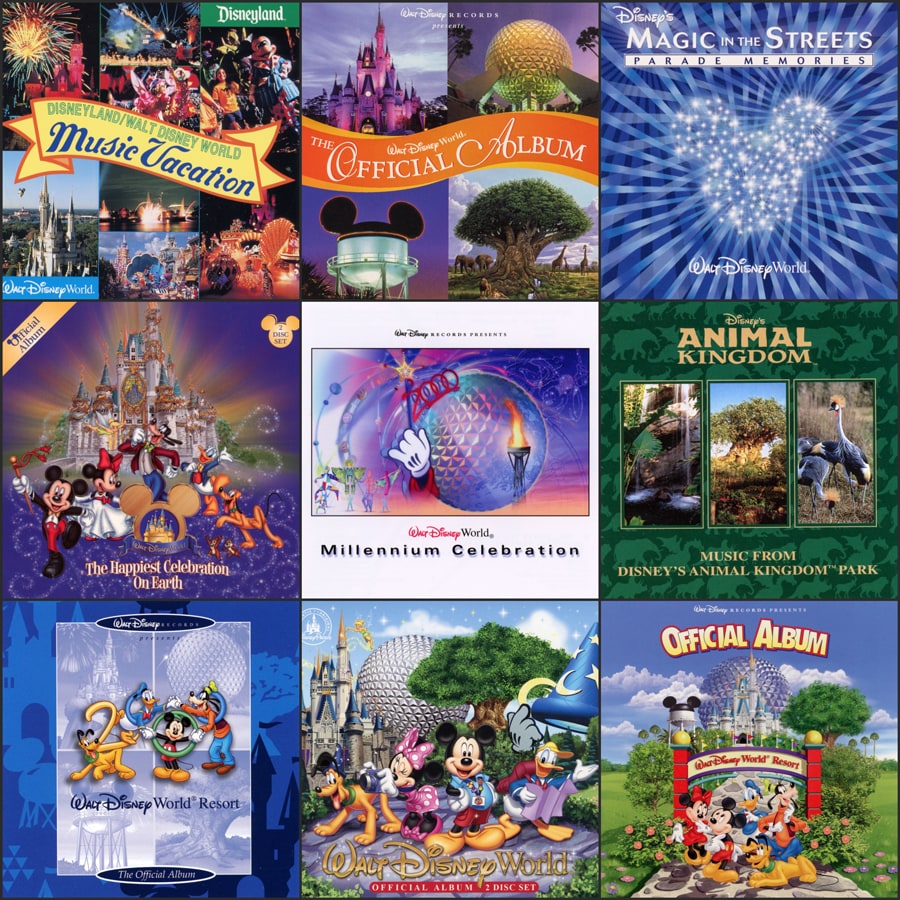The image depicts a collection of nine album covers, arranged in three rows and three columns, highlighting various Disney themes and parks. Each square-shaped album cover showcases iconic Disney characters and locations. The top left album is titled "Disneyland Music Vacation," featuring images of classic Disney characters. Adjacent to it is "The Official Album" of Walt Disney World, showcasing landmarks such as the Magic Kingdom Castle and Epcot Center. The top right cover, "Magic in the Streets: Parade Memories," displays a glittering Mickey Mouse head resembling a disco ball. The middle row includes "The Happiest Celebration on Earth Album" with Mickey, Goofy, and other characters in front of the Magic Kingdom Castle, a "Walt Disney World Millennium Celebration" album, and an album specifically for "Disney's Animal Kingdom" featuring photographs of animals like crest-bearing cranes and possibly an ape. The bottom row comprises a Walt Disney World Resort album with more cartoon characters, a center album highlighting Epcot Center and various iconic Disney elements such as the Fantasia hat, and an "Official Album" showing the gate leading into Disney World surrounded by characters. The shared emphasis is on Mickey Mouse and other beloved Disney characters across different park-themed albums.